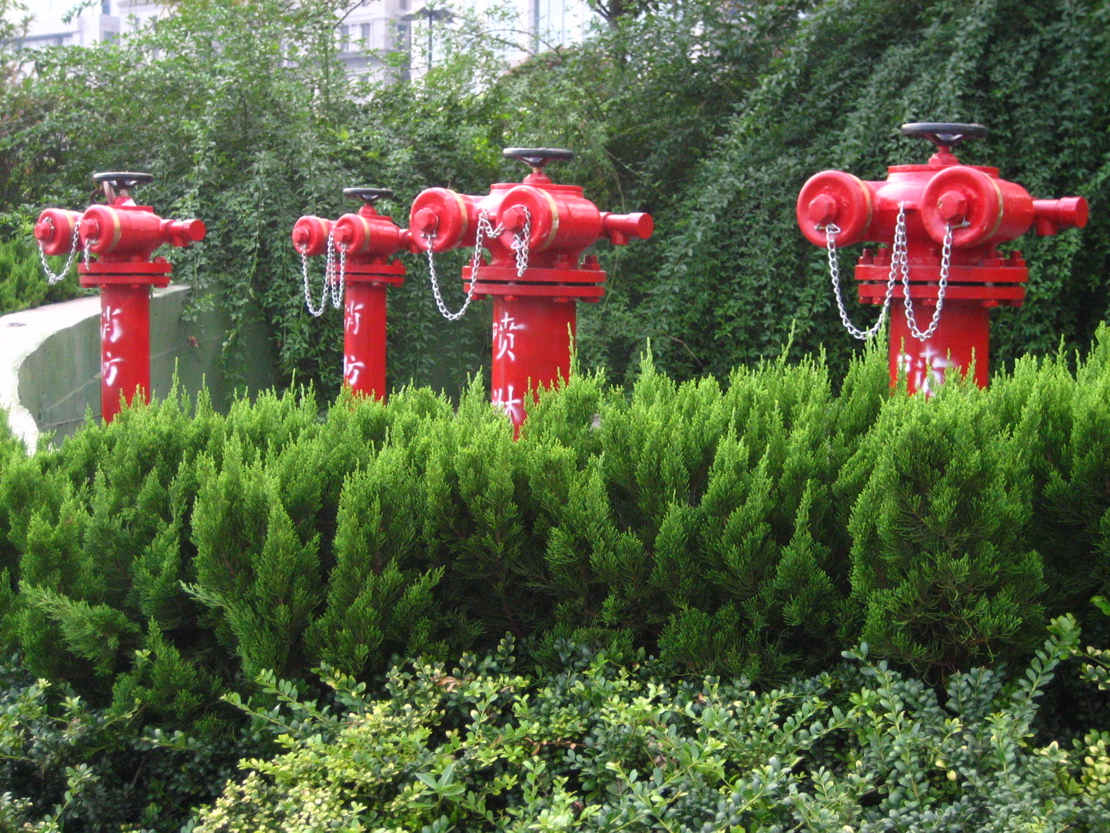This daylight photograph captures four tall, red fire hydrants standing behind a concrete wall adorned with green ivy. Each hydrant features a black crank at the top and a silver chain hanging in front of two nozzles. White lettering in a foreign language is visible on the hydrants. In front of the hydrants, a variety of green vegetation is present—bright green bushes and smaller plants with lighter green and white hues. Tall trees with long, green branches and an array of buildings are seen in the background, adding depth to the scene. The lush greenery partially obscures the concrete wall, contributing to the vibrant, natural ambiance of the outdoor setting.